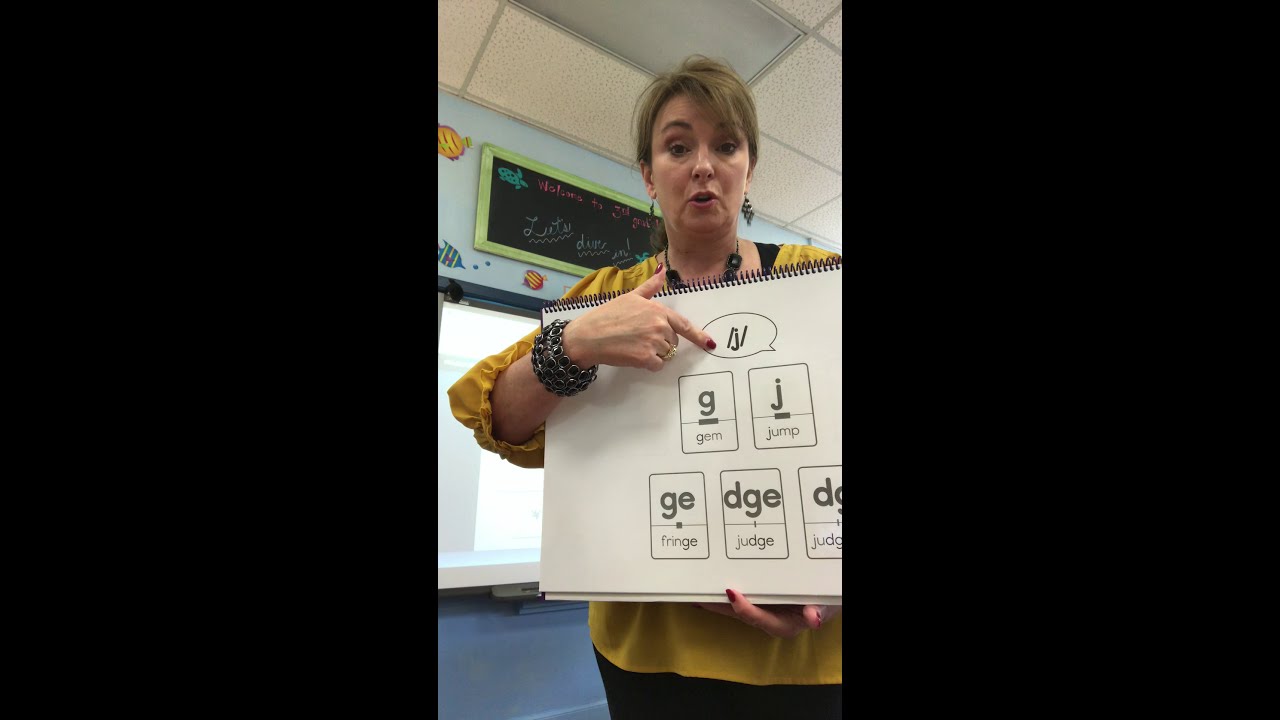In this detailed photo, a woman, presumably a teacher, is standing in a classroom setting. Her brown hair is neatly tied back, and she is adorned with chandelier earrings, a chunky necklace, bracelets, a billowy yellow shirt, and black pants. She is holding a spiral-bound presentation board in her left hand, which is positioned towards the camera. The board features educational content about the pronunciation and spelling of the /J/ sound. It includes the letters "G" with the word "gem" beneath it, "J" with the word "jump," "GE" with "fridge," and "DGE" with "judge." The board has five individual cards, and she uses her right hand to point at the letters and words, specifically focusing on the letters "G" and "J."

The backdrop of the scene reveals a classroom environment decorated with educational and decorative elements. Directly behind her is a blue wall covered with tropical fish images or decals, and to her left, a blackboard features welcoming messages written in chalk, including "Let's dive in" and "Welcome to the third grade." A computer monitor and what appears to be posters or projected images are partially visible. The ceiling has a suspended design with recessed fluorescent lighting, and small cardboard fish decorations are also visible, adding to the aquatic theme of the decor. This appears to be a screenshot from an educational video focused on teaching spelling and pronunciation to third-grade students.